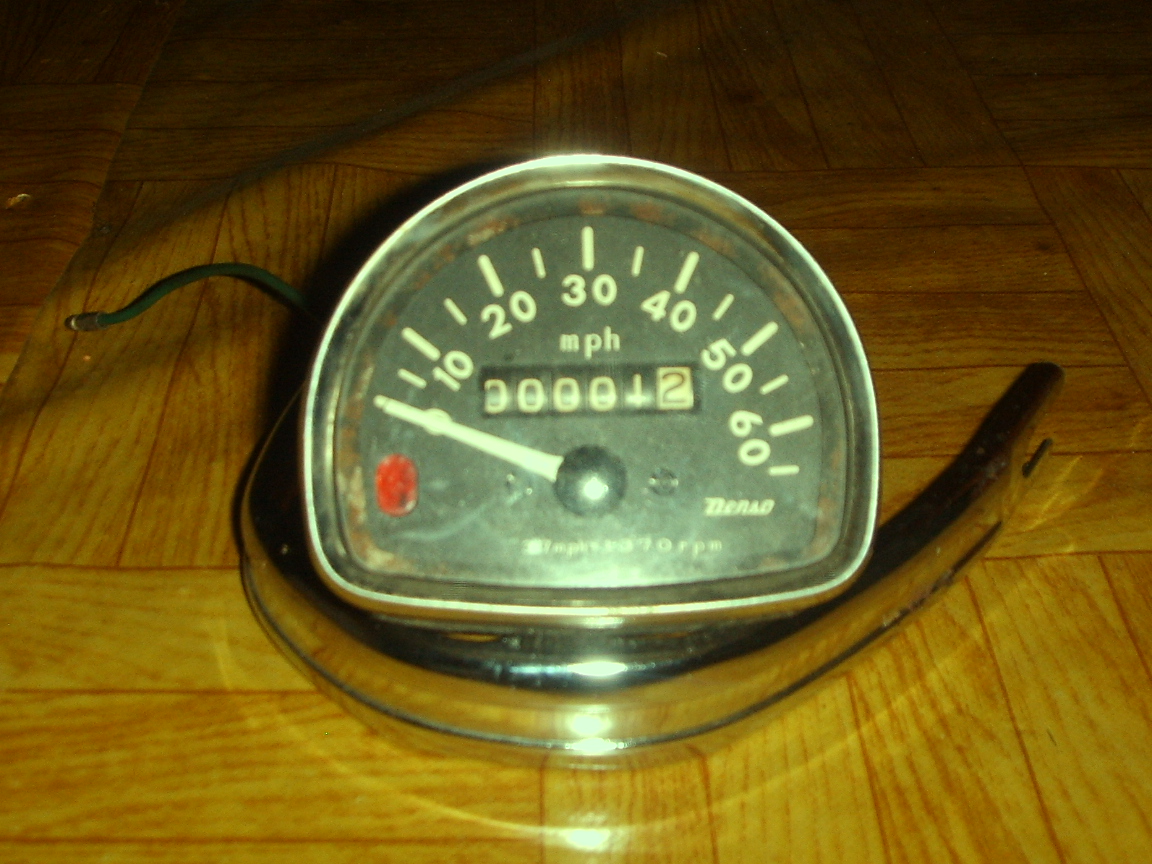In the image is a room with a light wooden floor. At the center, there is a bed featuring a gray and cyan color scheme, adorned with various rectangular patterns. A distinctive object in the scene appears to be an instrument for measurement. This instrument is adorned with metallic accents and houses a speedometer, which displays mileage. The speedometer's needle rests at zero, disconnected from its usual context. Below the gauge, the letter 'X' is visible. Just above the mileage, the letters "MPH" are printed in white. A black circle in the middle houses a light, and to the left, a red oval-shaped dot can be observed. The instrument is encased in a transparent covering, possibly made of plastic or glass, which reflects light slightly.